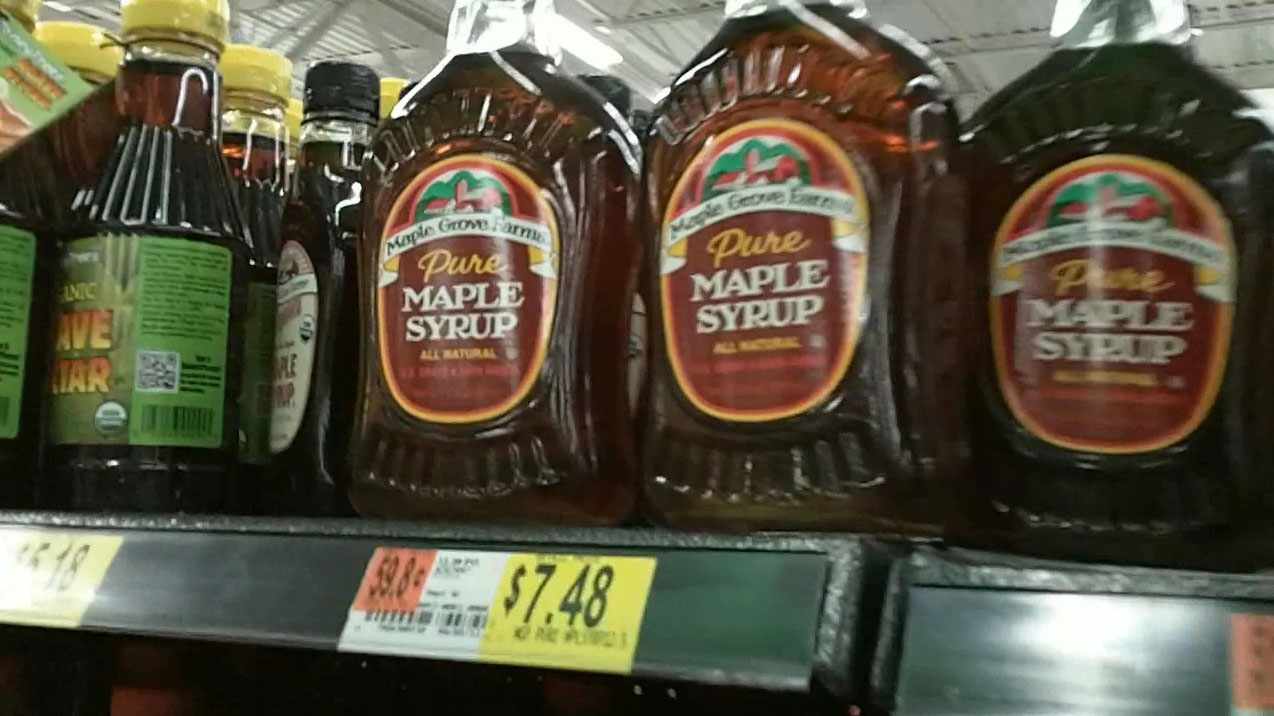This detailed and richly textured photograph, taken inside a grocery store that could be a Walmart, focuses on a shelf stocked primarily with bottles of Pure Maple Syrup from Maple Grove Farms. The clear plastic bottles, filled with brown, amber-colored syrup, feature labels with a green and red background depicting a farm scene. Prominent texts on the labels include "Pure Maple Syrup" in white, and "Maple Grove Farms" along with "All Natural." To the left of these bottles, another brand appears to offer agave nectar, identified by a green label and a yellow plastic cap, priced at $5.18. The price tag for the Pure Maple Syrup reads $7.48, and multiple price tags and product sizes are visible along the gray shelf. In the broader setting of the store, additional text and the top of the store are seen in the background, adding depth to the image's complex composition.